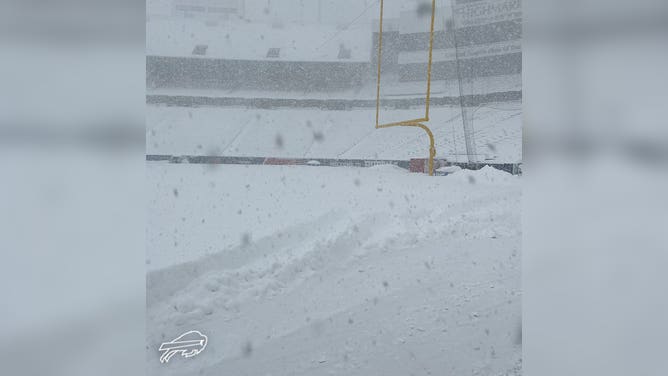In this detailed daytime outdoor photograph, a football stadium is completely buried under a thick blanket of snow, reaching several feet high with no visible footprints or people. The snow continues to fall heavily, evident from the numerous white particles – the snowflakes – captured in the image. A dark yellow football goalpost stands tall and is positioned towards the top right corner of the photograph, its distinct vertical sides and curved base easily discernible against the snowy field. The stadium, featuring multiple storeys and a high wall behind the goalpost, is almost entirely cloaked in white. A scoreboard, faintly visible, adds to the scene's authenticity. Despite the entire field being obscured by layers of snow, the photograph captures the essence of a heavily snow-laden football arena, with a goalpost as a key identifier amid the whiteout conditions.